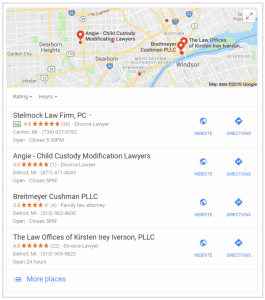This is a screenshot of a Google Maps interface displaying several law firms specializing in family law within the Michigan area. The map highlights regions including Dearborn Heights, Garden City, Windsor, and Dearborn. Below the map, detailed listings of various law firms are provided:

1. **Stelmach Law Firm, PC**:
   - Rating: 4.8 stars
   - Specialty: Child Service Lawyer
   - Location: Canton, Michigan
   - Contact: 734-927-9782
   - Operating Hours: Open, closes at 5:30 PM

2. **Angie, Child Custody Modification Lawyers**:
   - Rating: 5 stars
   - Specialty: Divorce Lawyer
   - Location: [Blurry section], Michigan
   - Contact: [Blurry section]
   - Operating Hours: Open, closes at 5:00 PM

3. **Brightmeyer Cushman, PLLC**:
   - Rating: 3.8 stars
   - Specialty: Family Law Attorney
   - Location: Detroit, Michigan
   - Contact: 313-962-8600
   - Operating Hours: Open, closes at 5:00 PM

4. **The Law Offices of Kirsten Irie Iverson, PLLC**:
   - Rating: 4.5 stars
   - Specialty: Divorce Lawyer
   - Location: Detroit, Michigan
   - Contact: 313-909-9823
   - Operating Hours: Open 24 hours

The image itself is small and somewhat blurry, with no photographic elements or people shown. It serves primarily as a directory for selecting family law attorneys in the specified region.